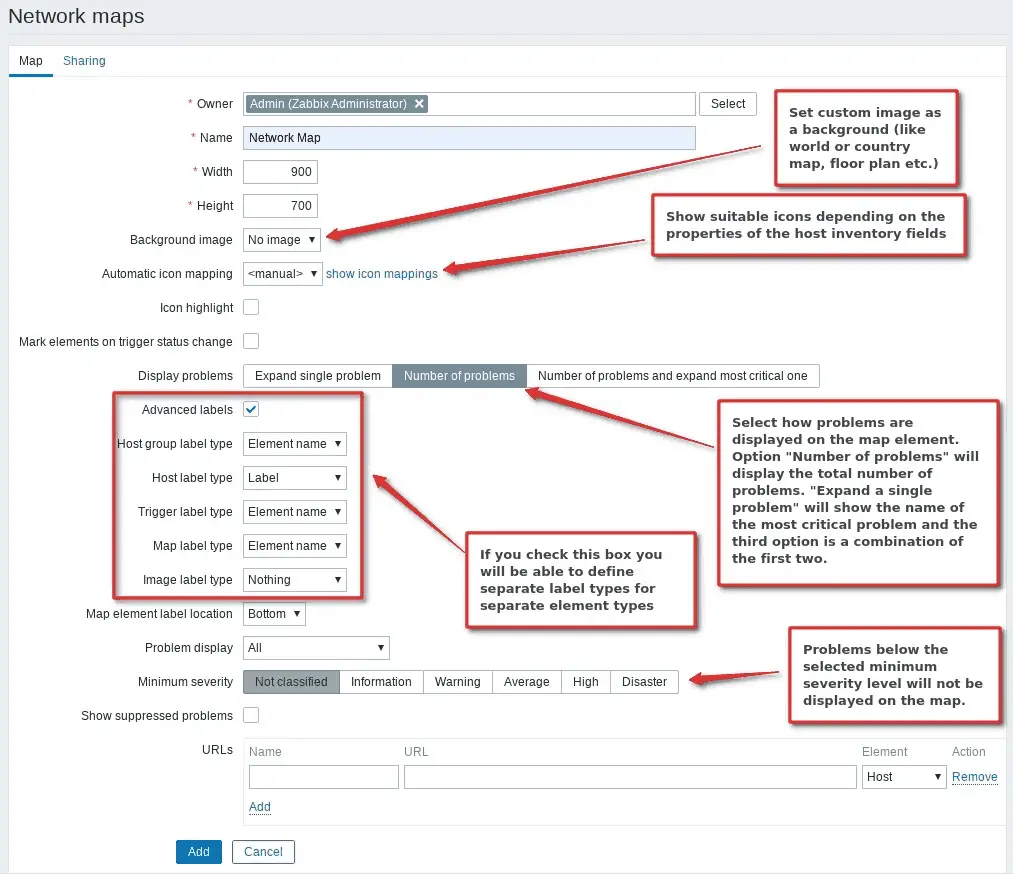This screenshot displays a program interface with a predominantly white background and text in black, interspersed with blue. It contains various sections, each highlighted with arrows connecting to explanatory text boxes. Notable elements include sections labeled "Network Maps," "Map Sharing," "Owner," "Owner Name," "Width," "Height," "Background Image," "Automatic Icon Mapping," "Icon Highlight," "Mark Elements," "Display Problems," "Advanced Labels," "Host Group Label Type," "Host Label Type," "Trigger Label Type," "Map Label Type," "Image Label Type," "Map Element Label Location," "Problem Display," "Minimum Severity," "Show Suppressed Problems," and "URLs." There are also functional buttons labeled "Add" and "Cancel."

Highlighted sections within the captured screen focus on the following:

1. **Background Image**: This section notes, "Set Custom Image as Background," suggesting options like a world map, country map, or floor plan.
2. **Automatic Icon Mapping**: Detailed as showing suitable icons depending on the properties of the host inventory fields.
3. **Number of Problems**: Options are provided to select how problems are displayed on the map element. Choices include:
    - Displaying the total number of problems.
    - Expanding a single problem to show the name of the most critical issue.
    - Combining both previous options to show a comprehensive view.

Further details include:

- **Advanced Labels through Image Label Type**: Checking a specific box enables defining separate label types for different element types.
- **Minimum Severity**: Problems below the selected minimum severity will not be shown on the map.

Overall, the screenshot captures a detailed setup and configuration interface for network mapping and problem display, allowing for customizable visualization and management of network elements.